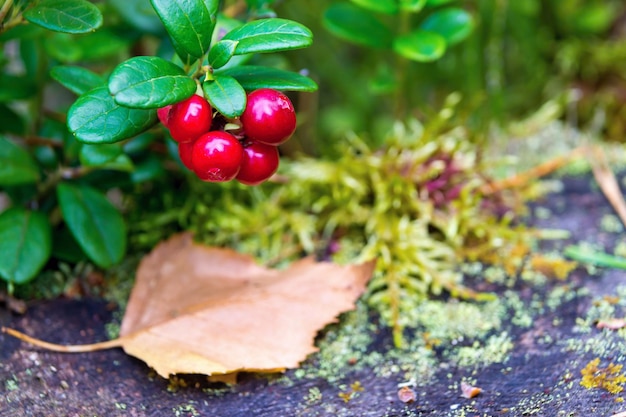This extreme close-up image features a vibrant green plant with almond-shaped leaves, accompanied by a striking bundle of bright red berries prominently positioned in the foreground. The berries, which appear to be bursting with juice, contrast sharply against a single brown, frayed leaf lying beneath them, which faces towards the right of the frame. To the right of this brown leaf is a mix of additional green and purple foliage. The image is characterized by a low depth of field, making everything except the central left part of the frame out of focus, resulting in a pleasing bokeh effect. The ground beneath the foliage appears gritty and dark. Off to the right, additional, out-of-focus plants blur into the background, softly outlining the scene.